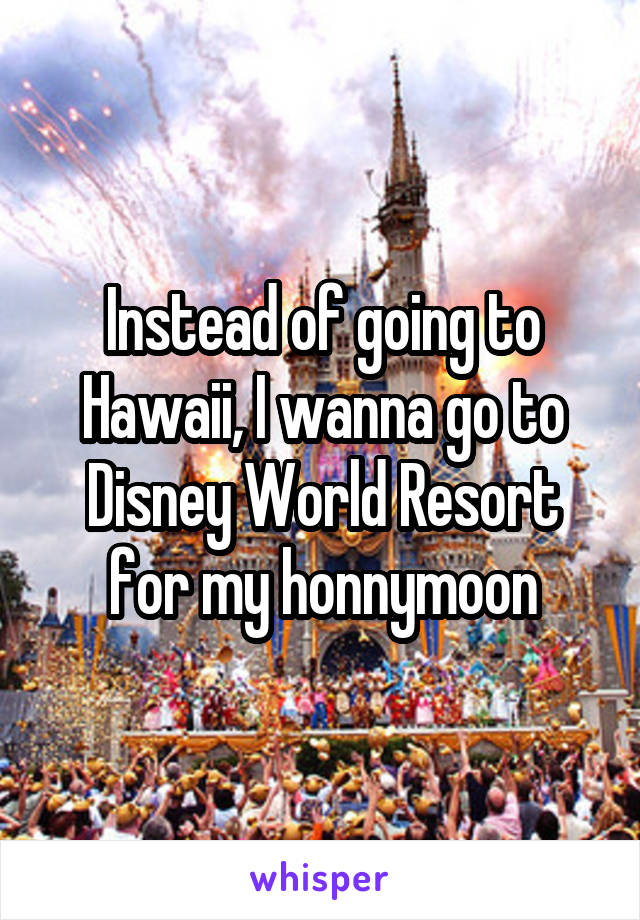The image is a full-color photograph taken outdoors during an overcast daytime, featuring Disney World's iconic castle as the central focus. Large white text outlined in black across the center reads, "Instead of going to Hawaii, I want to go to Disney World Resort for my honeymoon," with the word "honeymoon" misspelled as "honny moon." The castle is framed by a sky filled with fireworks, each leaving trails of dark smoke, and scattered clouds. At the bottom, a dense crowd with raised arms faces the stage, where Disney characters are lined up, surrounded by confetti, balloons, and banners in yellow and blue. The image quality is low, lacking detail, and includes a tree to the bottom left and some blue rooftops. The very bottom features a white banner with the word "whisper" written in purple lowercase letters.